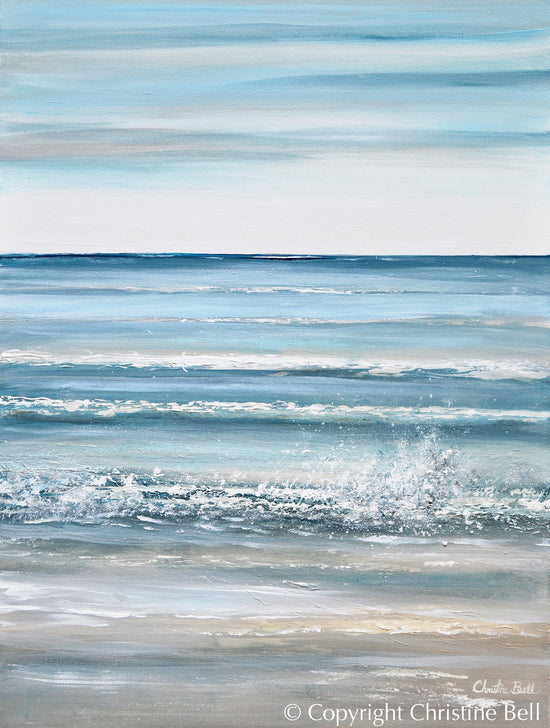This detailed acrylic painting captures a lifelike beach scene where the ocean meets the shoreline. Dominated by tones of blues and grays, the scene focuses closely on the water-covered sandy beach, with waves crashing and splashing along the shore. The white foamy crests of the waves are prominently depicted, extending towards the horizon where the water transitions from turquoise to a deep dark blue. Above the horizon, the sky fades from nearly white at the water’s edge to a mix of blues, pinks, and tans in the clouds. The painting is signed "Christine Bell," both in text and a handwritten signature, along with a copyright notice in the lower right corner.